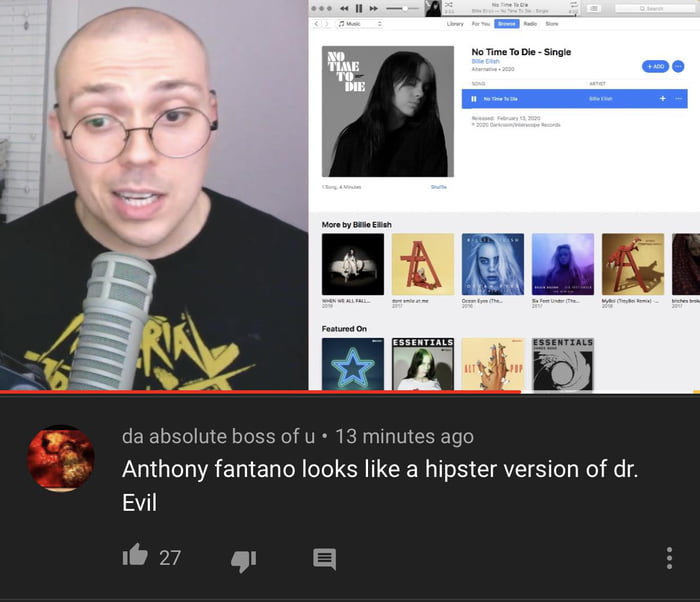This screenshot captures a YouTube or music app interface featuring a man speaking into a microphone. Dominating the left side of the screen is a large image of the man, who is wearing glasses and has a distinct appearance with one green eye, one brown eye, and one black eye. He is dressed in a black shirt emblazoned with yellow letters and has a partially bald head. 

On the right side, there is an album cover titled "No Time To Die," indicating it is a single by Billie Eilish. Below this, a blue bar with text too small to read spans across, followed by the section titled "More by Billie Eilish," displaying six of her other albums in a row. 

Further down is the "Featured On" section, showcasing four different boxes. 

At the very bottom, a black bar houses a comment section. The comment is from a user with the profile picture of a red circle and the username "the absolute boss of you," posted 13 minutes ago. The comment reads, "Anthony Fantano looks like a hipster version of Dr. Evil." Accompanying this comment is a thumbs-up emoji with 27 likes, a thumbs-down icon, a reply option, and a menu symbolized by three vertical dots.